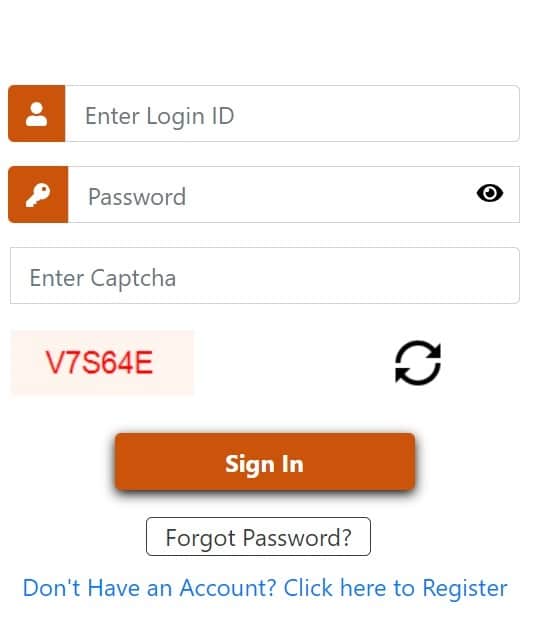The image illustrates a login screen for an account with a clean white background. At the very top of the screen is a square logo in a reddish burnt orange shade, featuring a white user icon. To the right of this logo is a light gray text box labeled "Enter Login ID."

Beneath the login ID field is another reddish burnt orange square, this one displaying a white key icon. Directly right of this square is a gray text box labeled "Password," with an eyeball icon at the far right, allowing users to reveal their password for verification.

Further down, the screen prompts users to "Enter CAPTCHA" with a corresponding CAPTCHA text box displaying the code "V7S6 4E." A refresh button is located to the right of the CAPTCHA box, enabling users to request a new code if the current one is difficult to read.

At the bottom of the screen, there's an orange "Sign In" button followed by a "Forgot Password" button. Below these options, there is an invitation for new users with a "Don't have an account? Click here to register" button.